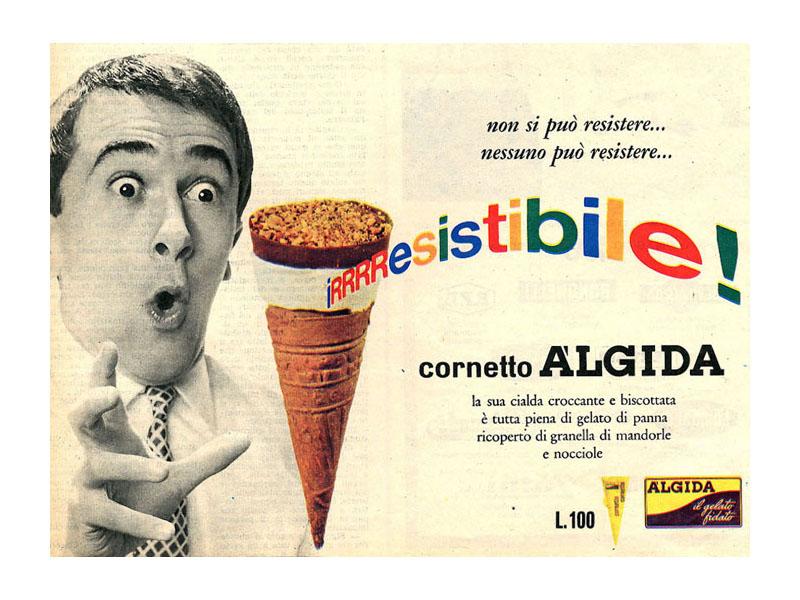This image depicts a retro poster advertising a Cornetto ice cream cone. On the left side, there's a black and white photograph of a light-skinned man with short, dark hair, wide eyes, and an 'ooh' expression on his open mouth. His right hand is extended in front of him as if he's about to grab something. He is dressed in a white collared shirt with a black tie featuring a diamond-like pattern. 

To the right of this image, there is a detailed illustration of an ice cream cone with a vanilla ice cream scoop covered in a chocolate coating and sprinkled with nuts. Above the ice cream cone, there are two lines of black text in a foreign language, possibly French or Italian. 

Emerging from the white ice cream layer on the right is the word "irresistible" in multicolored letters, starting small and increasing in size, ending with a green exclamation mark. Beneath this, in the bottom right of the poster, the brand names Cornetto and Algida are prominently featured in black text, along with additional lines of foreign text. There's also an emblem in the bottom right corner with further text that's too small to decipher clearly. To the left of this emblem, there’s a symbol that resembles a cone in a yellow wrapper accompanied by the text "L-100" in black.